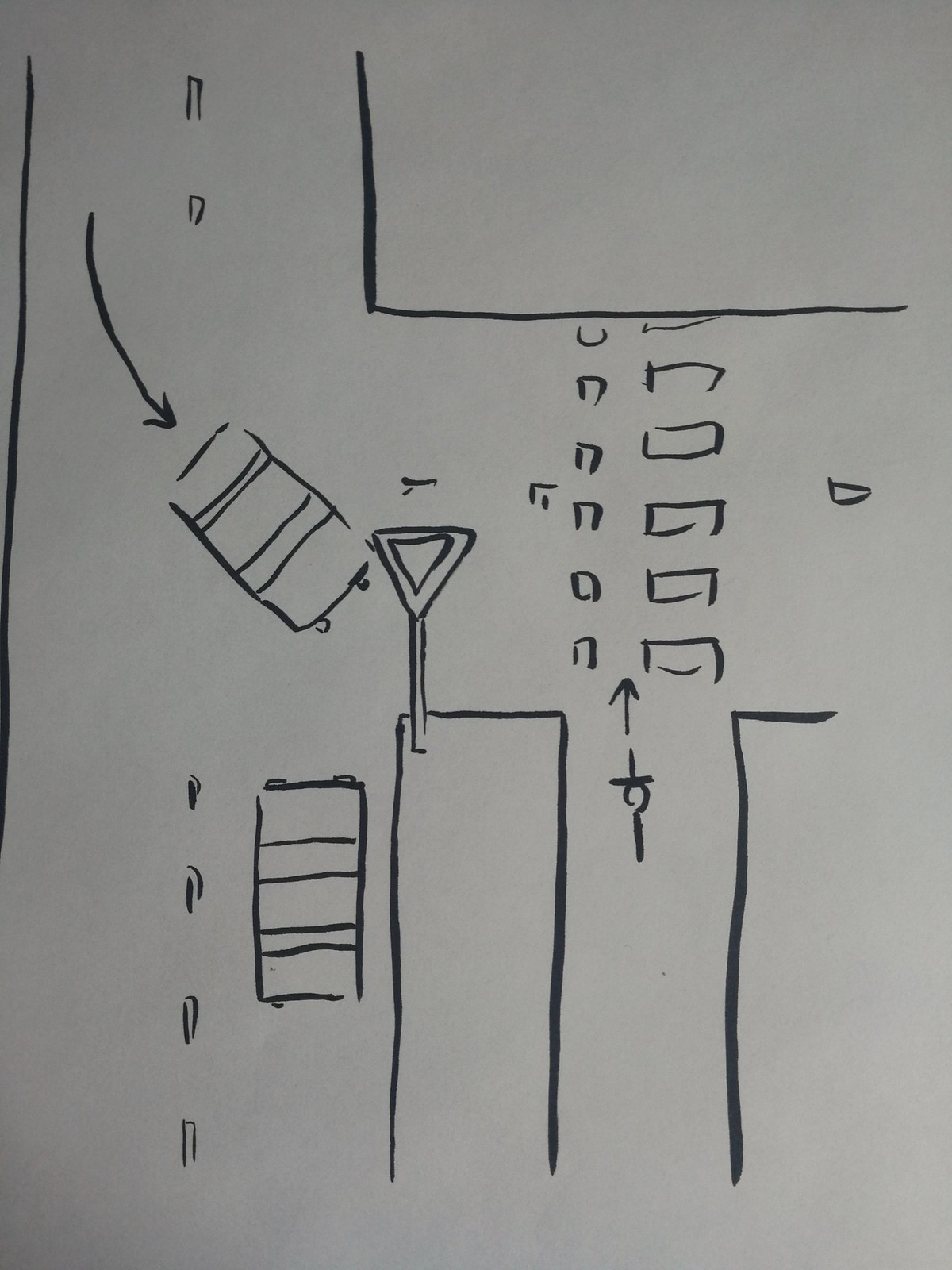This image depicts a whiteboard filled with black marker drawings, resembling a technical schematic or conceptual diagram. In the upper right corner, there's a densely shaded black rectangle segmented by a diagonal line running from the left-middle to the right edge. Adjacent to this blackened area, there are two U-shaped forms: one resembling an upside-down U almost forming a rectangle and a smaller U-shape facing the opposite direction.

An arrow pointing downward leads to a rectangular object resembling a battery, identifiable by two horizontal stripes and electrodes at the top. This battery is directed towards a yield sign, uniquely shown with a smaller yield sign nested inside it. The yield sign is mounted on a post, which connects to an open three-sided rectangle below it.

Next to this open rectangle lies another battery, marked similarly with two electrodes at the top and two horizontal stripes in its lower half. Four three-quarter rectangle shapes extend downward from this battery, aligned vertically along the bottom of the image.

Six small vertical rectangles, each with a block-formed letter U beneath them, are placed near the open-sided rectangle. To the right of these small rectangles is a tiny triangle shape. On the lower right section of the image, there appears to be a cross-like symbol with a circle around its center and an arrow pointing upwards. This symbol is nestled between another rectangular element depicted with only two sides.

Overall, the whiteboard is intricately covered with various shapes and symbols, possibly representing an electrical circuit or another technical design.